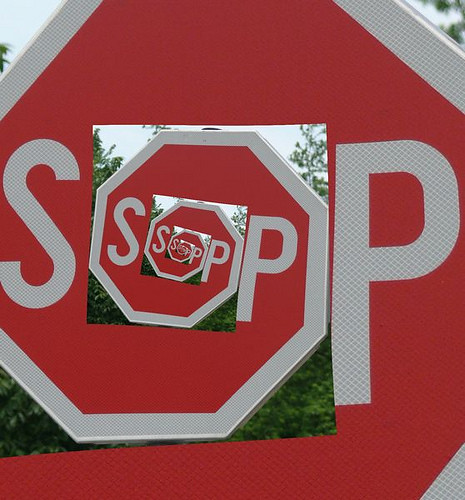The image is an edited, surreal depiction of a stop sign, transformed into a mesmerizing spiral that draws the viewer's eye into its center. The iconic red octagonal shape and large white letters "S" and "P" are repeatedly visible, curling counterclockwise into the center, giving the illusion of an endless loop. Each segment of the spiral mirrors the "S" and "P" of the stop sign, creating a fractal-like effect that makes the sign appear as if it's infinitely folding into itself. Despite this intricate alteration, the background scenery remains distinct, showcasing a bright blue sky dotted with green trees, grounding the surreal spiral in a familiar environment. This fascinating, seemingly impossible piece of art likely involved sophisticated computer software, enhancing the depth and captivating nature of the image.